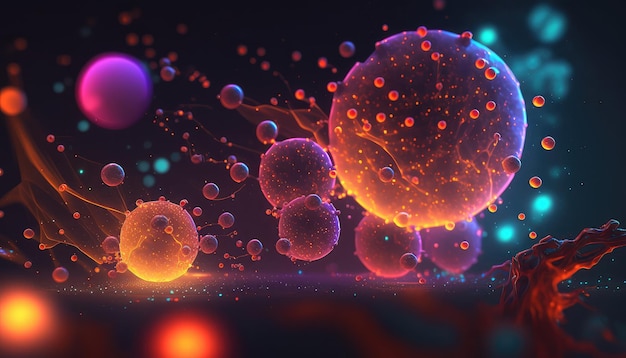This rectangular landscape image, almost twice as wide as it is tall, presents an otherworldly scene that could be interpreted as either a molecular landscape or a cosmic expanse. Set against a dark background that transitions from deep black to a dark blue on the right, the composition is dominated by an array of bubble-like spheres floating in an open space. The largest sphere is positioned slightly above and to the right of center. It features a predominantly lavender-purple hue with an orange-tinged lower left side, suggesting illumination from a light source situated at the lower left of the frame.

Adjacent to the largest sphere, particularly to its left and below, are four smaller spheres, each about half its diameter. These spheres share a similar purple-violet coloration. Additionally, another sphere of comparable size to these smaller ones is found to the left but exhibits a more pronounced orange tone.

In the lower left corner of the image, a bright orange sphere with a red rim resembles distant headlights, adding an intriguing focal point. This motif reappears elsewhere in the lower left part of the image, accompanied by numerous smaller spheres that populate the scene, many displaying shades of purple and violet.

On the right side of the image, faint aqua-colored lights appear in the distant background, further enriching the scene with their subtle glow. The entire landscape is interspersed with countless tiny spheres, contributing to the overall impression of an infinite, floating expanse. Whether depicting the molecular intricacies of matter or the vast, enigmatic depths of outer space, the image captivates with its mysterious and ethereal beauty.